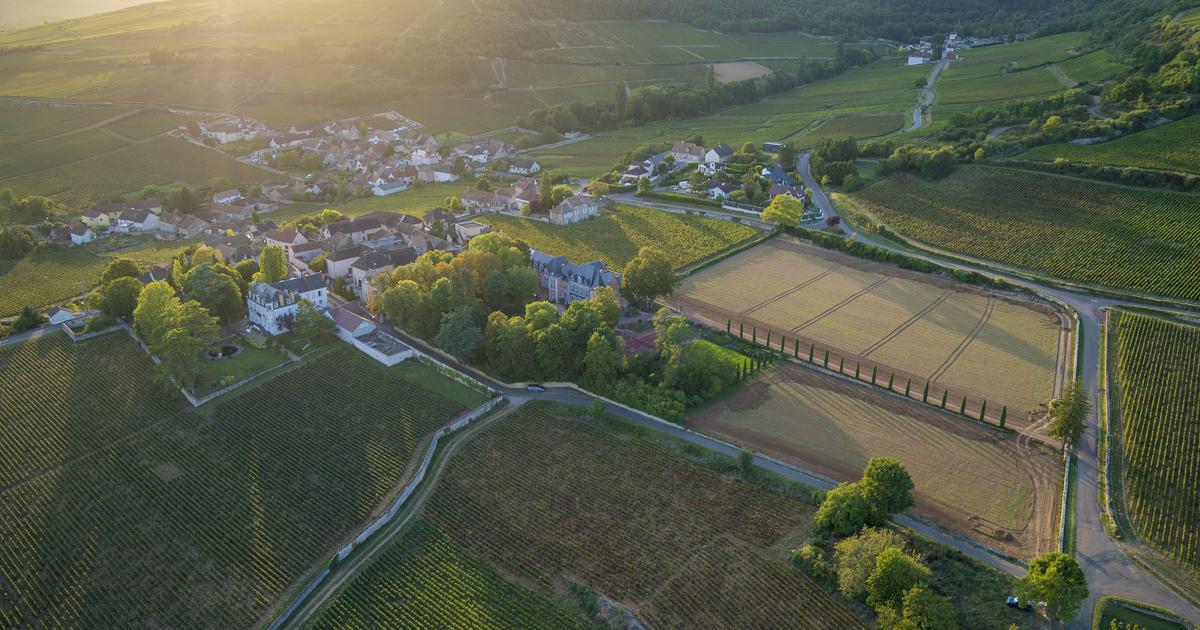In this picturesque aerial view of a countryside village, possibly in the United States or Europe, the lush green landscape of trees, grass, and fields dominates the scenery. The image, captured during either sunrise or sunset, is bathed in a warm, golden light, with sunbeams stretching across the terrain. A network of roads crisscrosses the village, converging at a central large building surrounded by smaller structures. These roads connect the town to the outskirts and beyond. Among the vibrant green meadows and grasslands, small white houses with darker roofs dot the landscape, gathering in clusters that suggest either a small town or an interconnected township with premium residences. Notably, there are two areas of ploughed brown earth, which stand out amid the greenery, possibly serving as playgrounds or fields awaiting cultivation. Cars can be seen traveling on the roads, emphasizing the village's connectivity and the gentle hum of daily life in this serene, verdant setting.